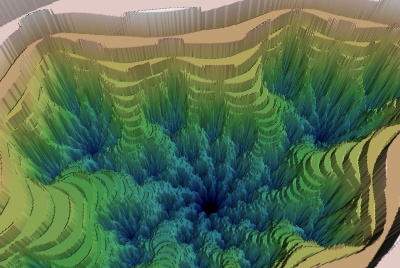The image appears to be a digital illustration resembling an underwater scene within an aquarium. It features various green and blue-hued plants and corals commonly found in such a setting. The view is from above, highlighting layers that resemble terraced land or step farming patterns, creating a sense of depth. Around these central green plants, there's a mix of blue vegetation, suggesting a vibrant aquatic environment. The illustration has a textured, almost cavernous look with surrounding bands of brown and orange, possibly mimicking the sandy floors of an aquarium. The lighting is bright, fading into different shades of green and blue, enhancing the underwater illusion and evoking a tranquil, otherworldly atmosphere.